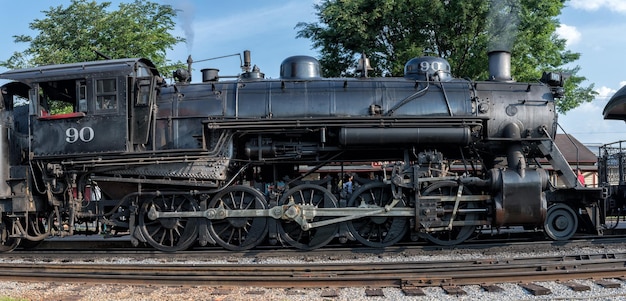The image captures a detailed side view of a vintage black steam locomotive with the number 90 emblazoned in white on its engineer cab. The locomotive, positioned on dark brown metal train tracks, occupies about 9% of the horizontally rectangular frame. The black steel machine exudes a striking presence with its cylindrical body and an array of intricate mechanical components, including large black metal wheels connected by light gray metal rods, and additional tubes and rods beneath the chassis. At the front, a small smokestack emits a plume of smoke, accentuating the historical essence of the train. A small platform juts out over the front wheel, adding to the locomotive's detailed architecture. The setting is outdoors on a clear, sunny day, with vivid blue skies dotted with light white clouds. The backdrop features lush green treetops and a prominent tree extending out of the frame at the top, providing a serene contrast to the imposing black locomotive. In the foreground, white rocks and small boards peek out from beneath the tracks, emphasizing the rustic and open-air scene.